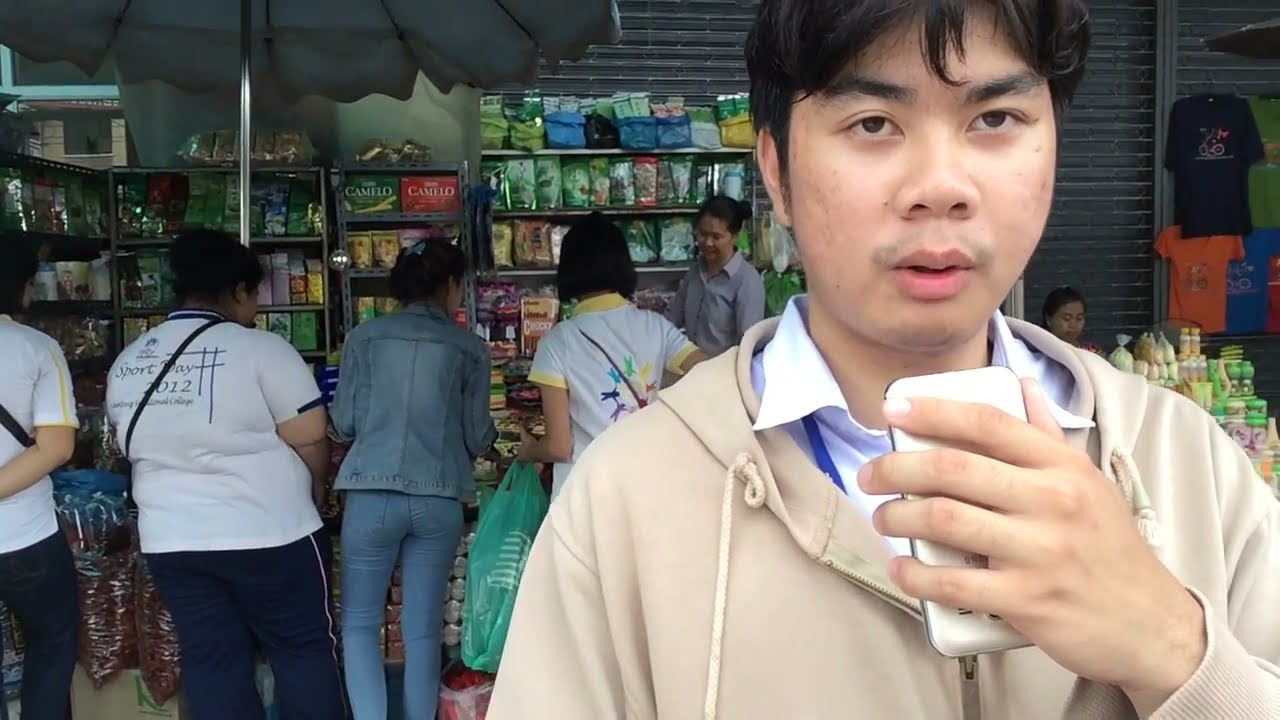In this detailed photograph, we see an Asian man prominently positioned in the foreground, slightly to the right. He has medium-length black hair and a bit of stubble around his mustache area. He's wearing a beige or tan zip-up hoodie over a blue shirt, which might also feature a blue stripe or a darker blue lanyard. In his left hand, he is holding a white smartphone. His body and gaze are oriented towards the 5 o'clock position, giving him a somewhat perplexed expression.

The setting appears to be a lively market or grocery store, with a variety of products displayed on shelves and behind counters. In the background, we see multiple people with their backs to us; most are young women standing in a horizontal line. On the right, a woman in a white, yellow, and multicolored shirt stands out, while another woman in a denim jacket is situated to her left. Further left, there's a woman in athletic pants and a white t-shirt with graphics on the back. Additionally, a man in a blue shirt is behind the counter, possibly serving a customer. The scene also features various products, including t-shirts and food items, and even an umbrella on the left side. The overall atmosphere suggests a bustling and diverse market environment.